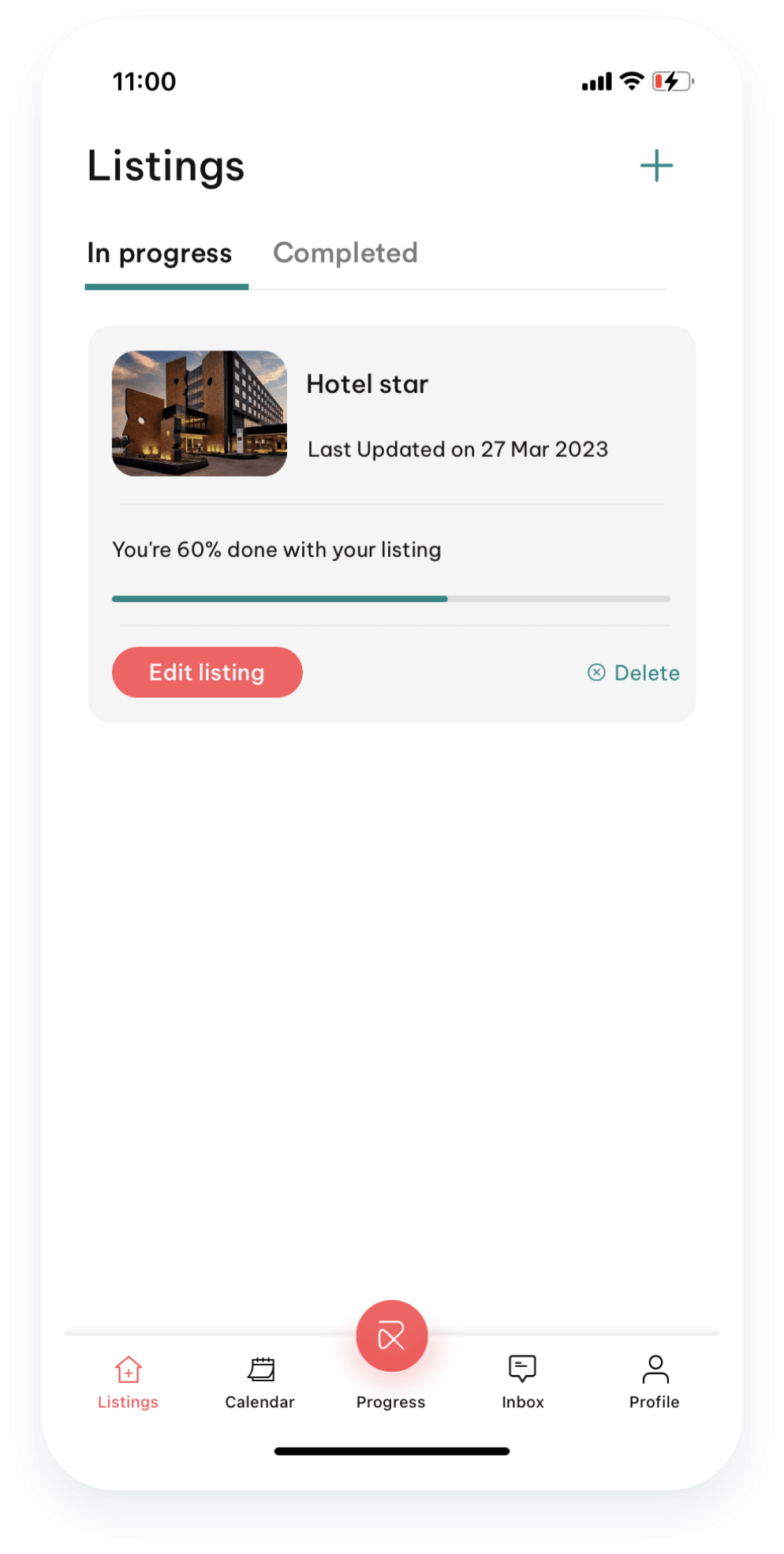The image is a screenshot of a mobile application screen with a white background, captured on a cell phone. At the top-left corner, the time is displayed as 11:00 in black lettering. In the top-right corner, the status bar shows four signal bars, a Wi-Fi connection symbol, and a battery icon with a red bottom indicating low power and a charging symbol.

Beneath the status bar, the word "Listings" appears in black on the left. On the right side, there is a gray plus button. Below this header, there are two tabs labeled "In Progress" and "Completed." The "In Progress" tab is in dark black print with a black or green underline indicating it is selected, while the "Completed" tab is in lighter gray and not selected.

Under the "In Progress" tab, there is one listing displayed in a gray rectangle. The listing is titled "Hotel Star," with a note indicating it was last updated on 27 March 2023. It shows that the listing is 60% complete, visualized by a progress bar with 60% filled in green and the remainder in gray. Below the progress bar, there are two buttons: a red "Edit Listing" button on the left and a green "Delete" button on the right. Additionally, there is an image of the hotel associated with the listing.

At the very bottom of the screen, there are navigation headings that read: "Listings," "Calendar," "Progress," "Inbox," and "Profile."